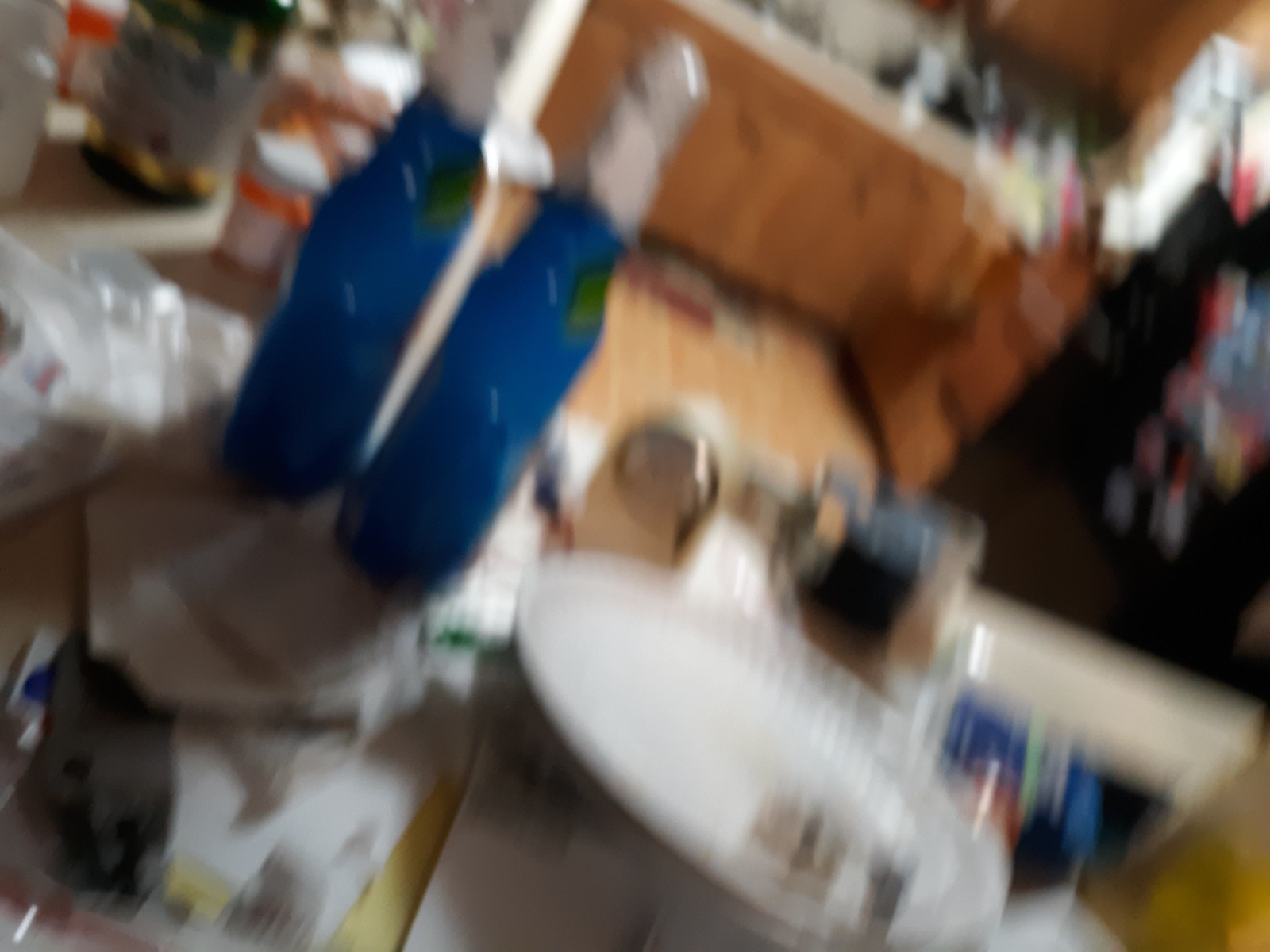This blurred photograph appears to have been taken with a camera in motion, resulting in a lack of sharpness and clarity. The image depicts a kitchen environment with visible countertops, cabinets, and what seems to be a refrigerator in the background. The lower portion of the image shows a cluttered table covered with various items, including what seems to be two blue bottles, several white ceramic plates, and scattered paper trash. Additionally, there are possibly one or more pill bottles among the items on the table. The upper half of the photograph features an array of kitchen cabinets, contributing to the overall impression of the space being a kitchen.